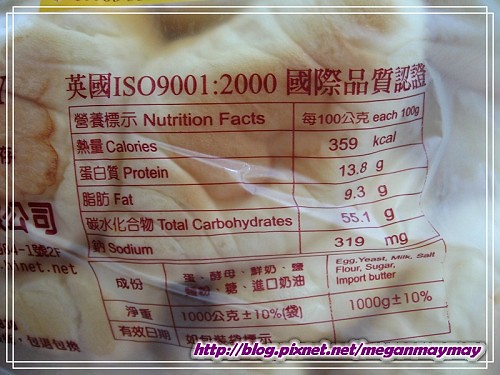This image features a plastic bag containing several pieces of croissant-like bread, prominently displaying the packaging and nutrition facts. The bread, cut into small chunks, is encased in a clear plastic bag, allowing a view of its texture and golden-brown color. The nutrition facts, printed in red ink, are primarily in Chinese with some key details translated into English, listing information such as calories, protein, fat, carbohydrates, and sodium content. On the left side of the bag, part of the product label is visible, including additional details in Chinese and a web link. In the bottom right corner of the image, there is a watermark, indicating the source of the photograph.